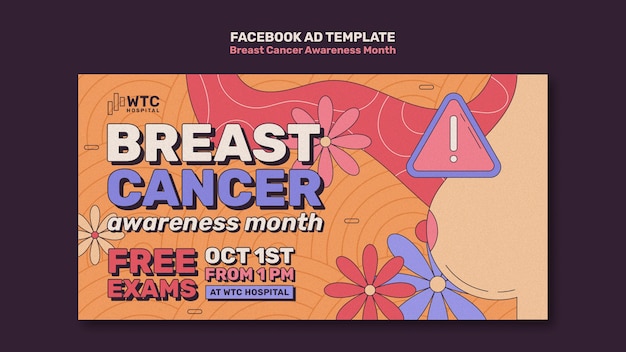This image is a digital screenshot, likely from a tablet or laptop, displaying a Facebook ad template focused on Breast Cancer Awareness. The ad features a black border and a central design. At the top, in all caps white text, it reads "FACEBOOK AD TEMPLATE." Below this, in smaller, pinkish text, it says "Breast Cancer Awareness Month." Further down, the text "WTC Hospital" is displayed prominently. 

The background features a combination of floral designs and non-filled curved rainbows, adding a sense of vibrancy. On the right side of the ad, there is a cartoon depiction of a woman's breast with a red triangle, outlined in purple, and a white exclamation point in the center, symbolizing alertness or caution. 

The floral elements are colorful, showcasing yellow, pink, red, and purple flowers that resemble daisies, enhancing the visual appeal and making the ad eye-catching. The main text of the ad emphasizes Breast Cancer Awareness Month and invites viewers for a free exam on October 1st at 1 PM at WTC Hospital.